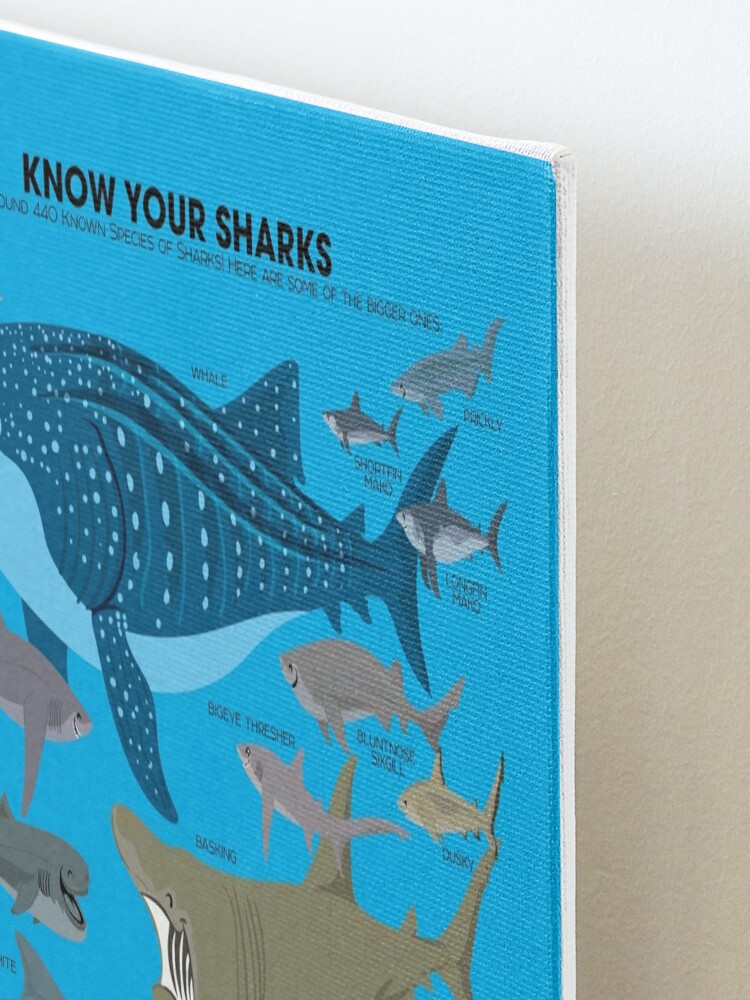The image displays a poster with a white border and a blue background, angled slightly. At the top, black text reads "Know Your Sharks" and underneath it states, "440 known species of sharks, here are some of the bigger ones." The poster features various cartoon sharks, each smiling, scattered around the main graphic. In the center, there is a large, blue whale shark, adorned with light blue spots and a lighter blue belly. Surrounding the whale shark are several other labeled shark illustrations: a shortfin mako to the right, a basking shark at the bottom right, and depictions of other species such as the bluntnose sixgill, longfin mako, dusky, and boweye thresher. The entire scene is well-lit, accentuating the vibrant colors and playful designs of the shark illustrations.